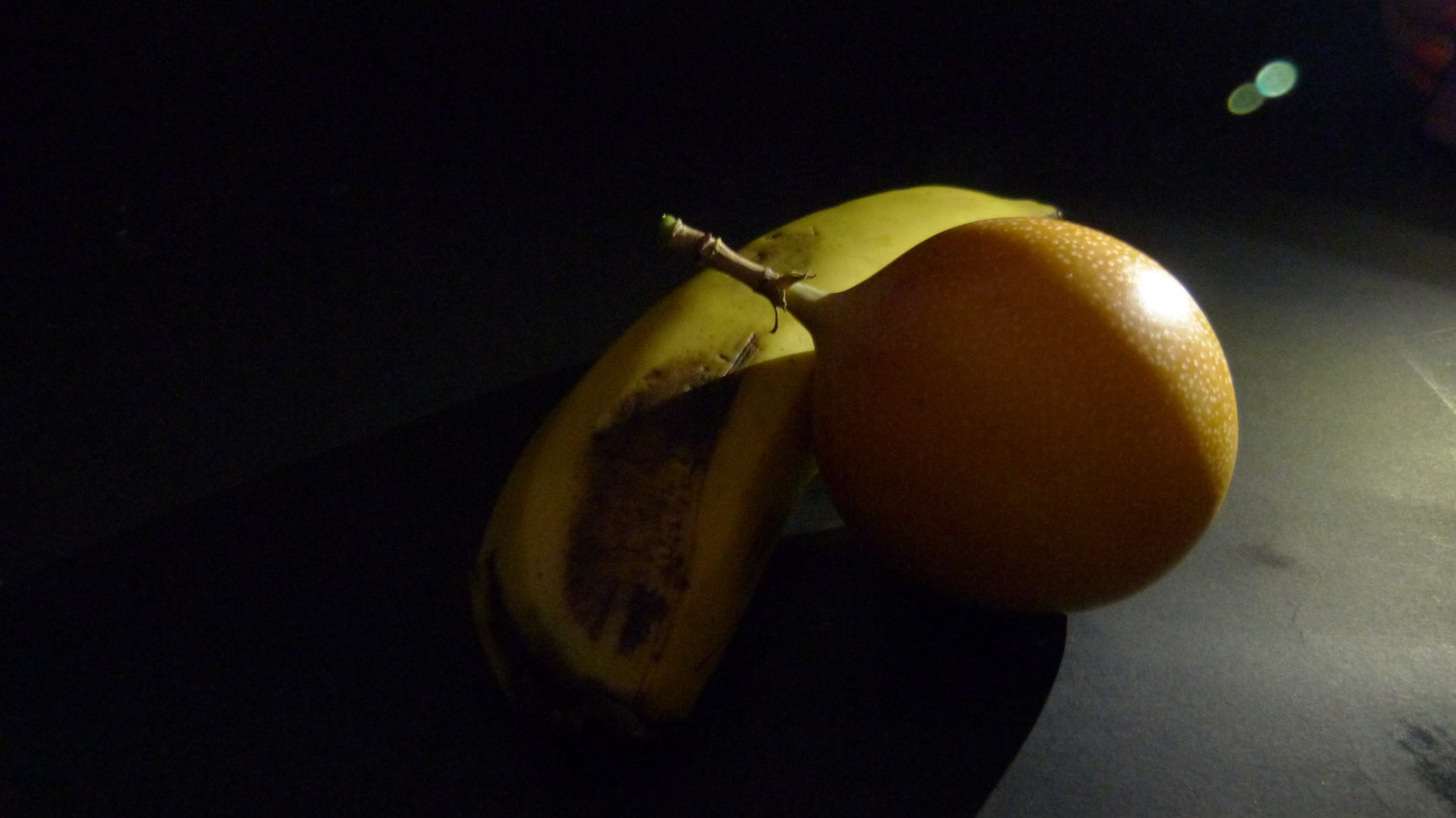A captivating artistic photograph in landscape orientation features a dark background that contrasts sharply with the illuminated surface, which appears gray or white. Central to the composition are two distinct fruits. One is a banana, atypically short and stubby, missing a defined tip or end. A large brown stain runs from the bottom center upwards, occupying over half of the fruit. The banana is positioned with its curve facing inward and the long edge stretching to the right.

Resting against the banana is an orange, vibrant in its round, orange form. The orange displays a curious characteristic: a noticeable brown stem with a green tip, suggesting it has recently fallen from a tree, which is uncommon for commercially presented oranges. The orange is tilted on its side, propped against the banana with its stem hovering above.

In the backdrop, two small green and light blue circles, possibly reflections from a camera, add an enigmatic touch to the scene. Additionally, a faint light in the right-hand corner gently illuminates the background, enhancing the depth and allure of this thoughtfully composed still life.